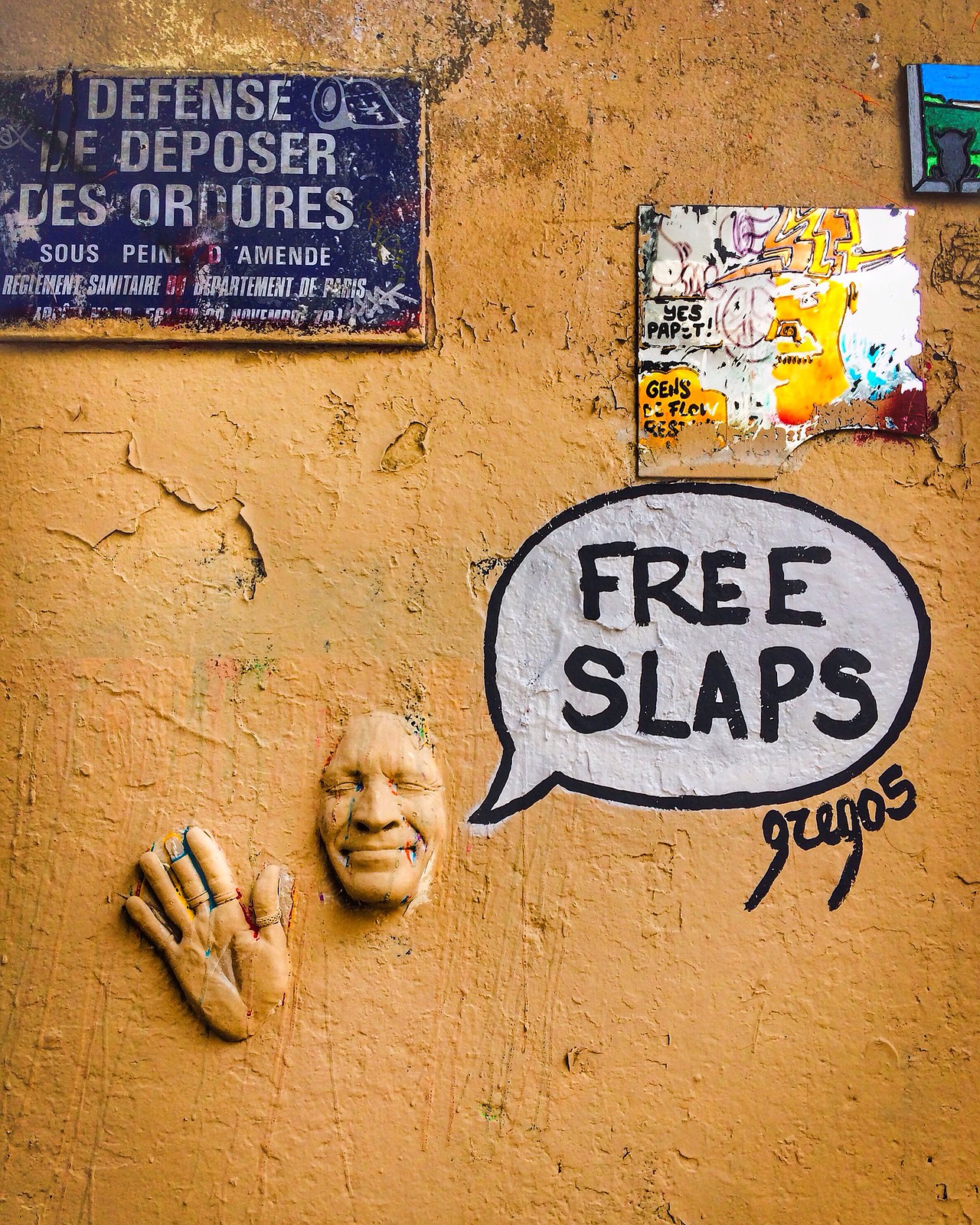The image depicts a weathered yellow stucco wall adorned with various signs and artworks. Dominating the scene is a detailed carving of a man's face, featuring a broad smile and a prominent nose, with an intricately sculpted hand extending outward. Above the face is a white speech bubble with black text that reads "Free Slaps." Below this, there appears to be a signature resembling "Grego 5." To the top left of the face, a blue sign with white lettering reads "Défense de Déposer des Ordres," hinting at French origins. On the right side of the composition, part of a colorful children's painting depicting a cat near a river is visible, adding a playful element to the weathered, sandy-toned wall. The overall scene suggests a mixture of urban art and signage, blending 3D elements and classic street art aesthetics.